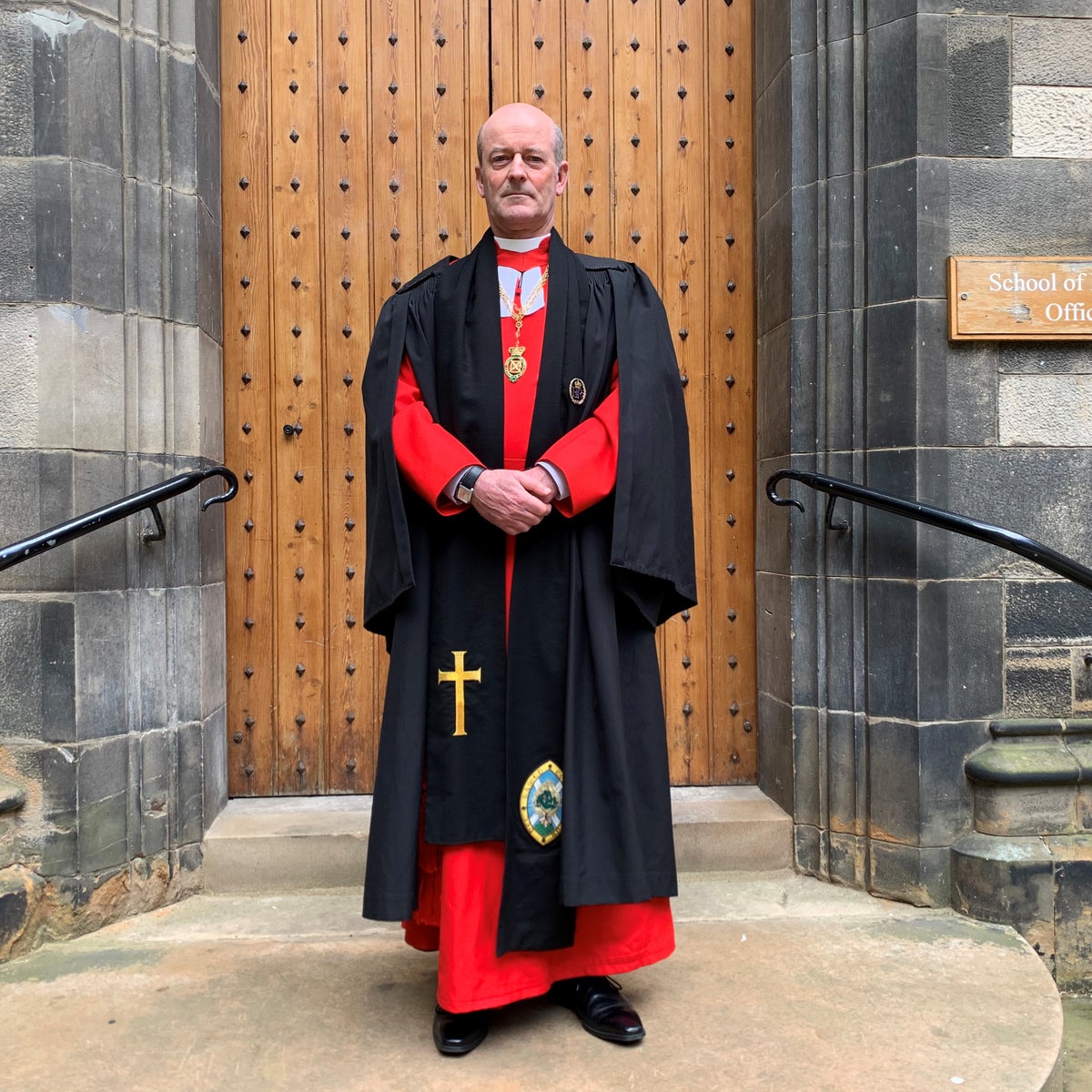The photograph captures an elderly, balding man, likely a Catholic clergy member, standing at the center of the image. He is dressed in a distinctive clerical outfit, consisting of a long red robe and a black over-robe adorned with an embroidered golden cross. A white clerical collar and a necklace add to his religious attire. The man, not smiling, gazes directly at the camera with his hands clasped in front of his stomach, also wearing a black wristwatch. He stands on stone steps leading up to a large, medieval-style wooden door, which features vertical slats and black metal embellishments. The door is framed by a stone building, and black metal railings curve around the steps. To the right of the door, a partially visible sign reads "School of" and "Office," suggesting a religious or educational institution.